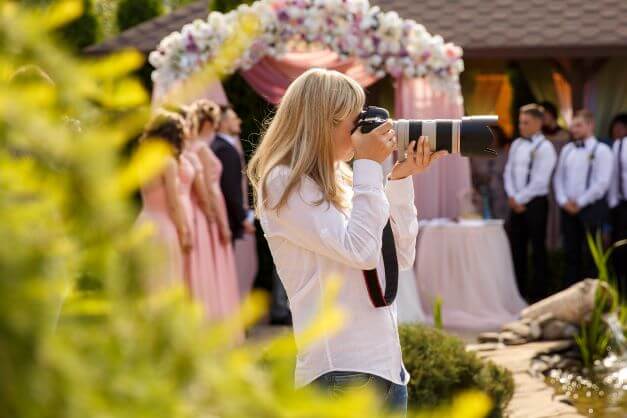In this vibrant outdoor daytime scene, a blonde woman dressed in a white long-sleeved shirt and denim jeans is seen holding a professional camera with a large black and silver lens, indicative of a wedding photographer. The wedding setting is elegantly adorned with an arch draped in pink cloth and topped with an array of pink and white flowers. Bridesmaids in light pink dresses and groomsmen in white shirts with black suspenders can be seen in the background, mingling near a garden and a gazebo, adding to the joyous and celebratory atmosphere.